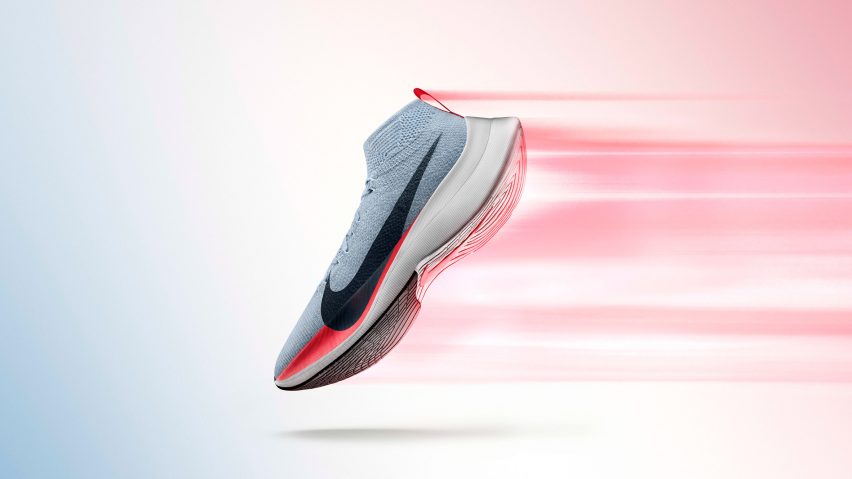This image shows an athletic Nike shoe prominently displayed against a light gray background, seemingly floating in mid-air with a subtle drop shadow beneath it. The shoe, which has a slip-on, sock-like design that fits snugly around the ankle, features a light gray upper made of breathable material. The shoe's front is adorned with a bold black Nike swoosh that extends down to its white sole, accented with touches of orange. A distinctive red tag is positioned at the heel. The shoe is angled diagonally, with the laces pointing to the left and the sole to the right. To emphasize motion and speed, the image is enhanced with red and white streaks of light emanating from the rear towards the arch, creating a dynamic effect as if the shoe is propelling forward.